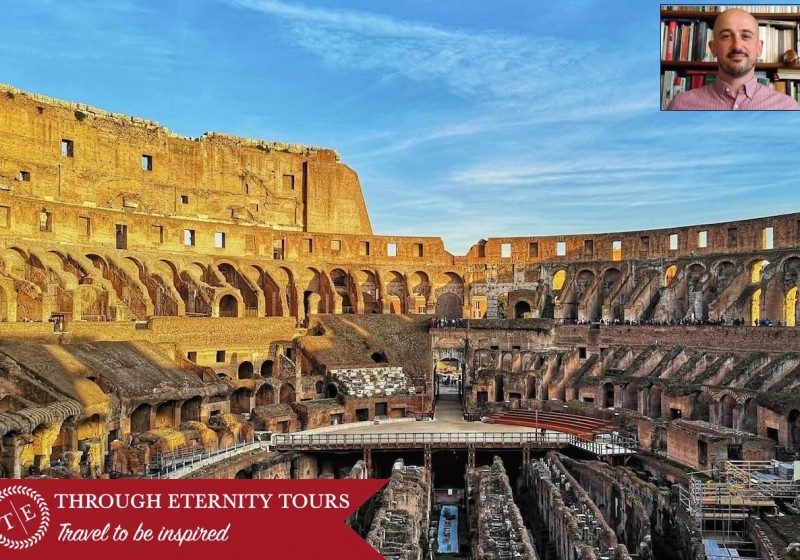The image portrays an engaging digital tour advertisement. In the top corner of the image, there's a photograph of a man with dark facial hair, wearing a reddish-pink shirt, standing in front of a bookcase filled with books, giving a scholarly vibe. The backdrop of the main image features a vibrant blue sky adorned with wispy white clouds. Dominating the scene are the ruins of what appears to be an ancient city square. The area is filled with weathered, crumbling buildings in brown and tan hues. At the bottom of the image, bright red and white text reads, "Through Eternity Tours: Travel To Be Inspired." The ancient cityscape, complete with scaffolding and a rough aesthetic, conveys an enduring allure of historical exploration.